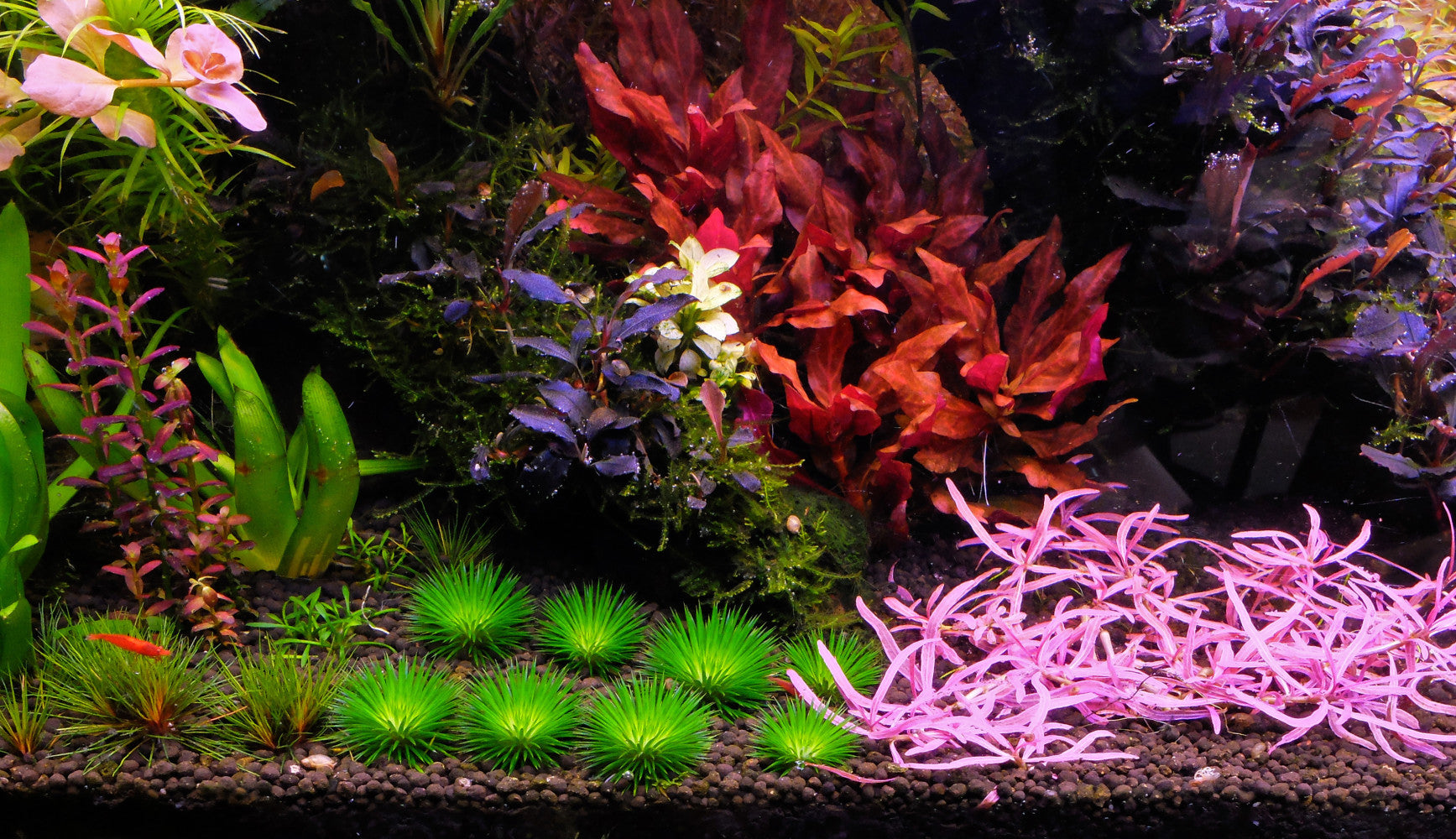The image depicts a vibrant and well-lit aquarium interior. The aquarium's bottom is lined with scattered brown pebbles, providing a natural base for a variety of aquatic flora. In the bottom left corner, a very small goldfish can be seen among the greenery. Various green plants, spiking outward in different directions, are positioned in the front middle and bottom middle areas, arranged in rows of eight. Intermingled with these are pink plants resembling noodles, adding a splash of color. 

The right side of the tank features a mix of purple flowers and orange elements, which could potentially be more fish or other aquatic flowers. In the upper left corner, there are pink flowers with green leaves. Central to the image are blue and red flowers, while the bottom right showcases pink, grass-like projections. The overall scene is one of diverse colors and textures, captured in sharp focus, especially towards the front, highlighting the intricate details of this aquatic habitat.